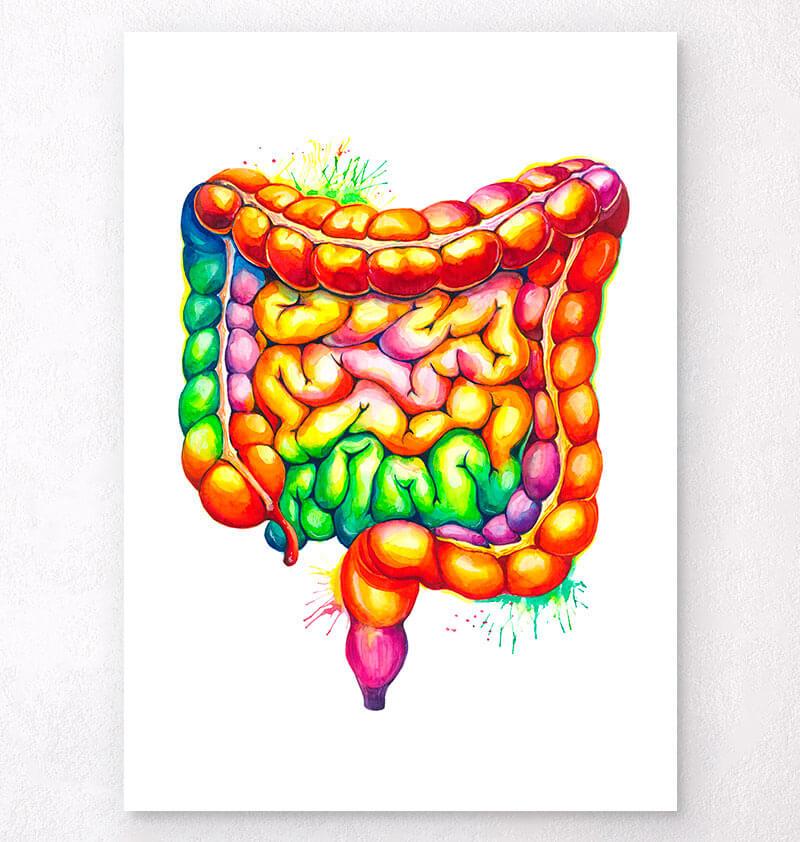The image is a detailed watercolor painting, rectangular in shape and poster-sized, depicting the human large and small intestines. The intestines are intricately illustrated, tightly wound together, and showcase a vivid array of colors, transitioning through orange, green, blue, red, pink, yellow, and purple. The large intestine dominates the left and upper portions, while the small intestine is nestled within, twisting and turning from left to right in a complex pattern. Notably, the tip of the intestine at the bottom is marked in purple.

The painting features distinctive watercolor splashes in the top left and bottom right corners, enhancing its artistic flair. The entire piece rests against a grayish-white background, with the edges artistically braided, adding a textural element to the composition. The colors of the intestines themselves fade seamlessly from one to another, creating a rainbow-like spectrum that adds to the visual intrigue and complexity of the artwork.